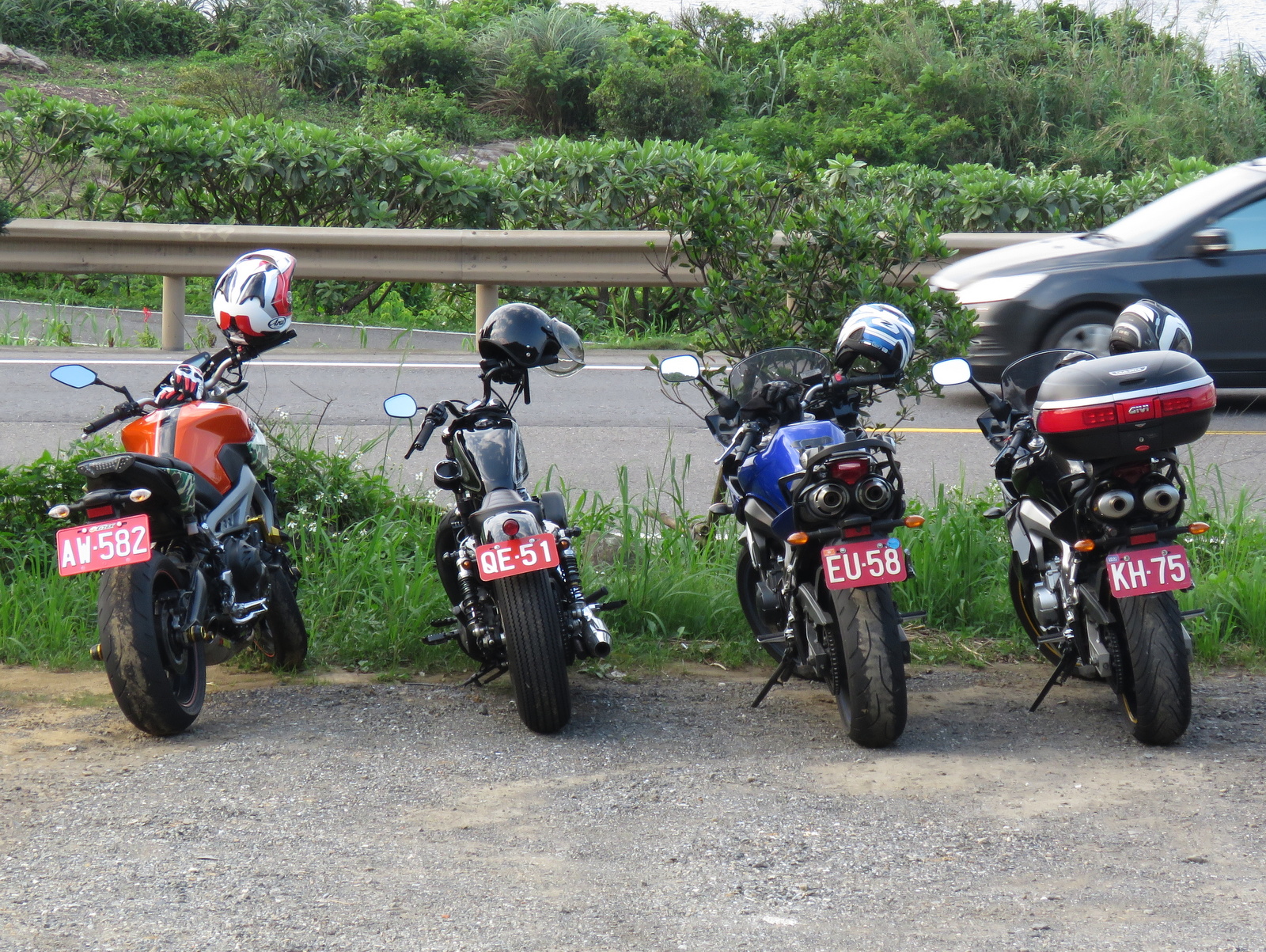The photograph captures a roadside scene on a cloudy day, showcasing four motorcycles neatly lined up on a gravel parking area with kickstands down. The motorcycles, all positioned with their rear wheels facing the viewer and evenly spaced, are adorned with helmets on their right handlebars. From left to right, the bikes are an orange motorcycle with a matching red and white helmet (license plate AW-582), a black motorcycle with a black helmet (license plate QE-51), a blue motorcycle with a blue and white helmet (license plate EU-58), and another black motorcycle with a black and white helmet (license plate KH-75).

In the foreground, there is a small grassy strip leading up to a road with a gray metal railing. The road features a yellow center line and white side markings, indicating an active roadway with a partially visible, moving black car on the right side, headed to the left. Behind the railing, there's a lush backdrop of green trees and bushes, hinting at a landscaped or natural setting beyond the road. The image suggests an outdoor stop or rest area adjacent to the road, with the motorcycles positioned on a gravel pavement, ready for the journey ahead.